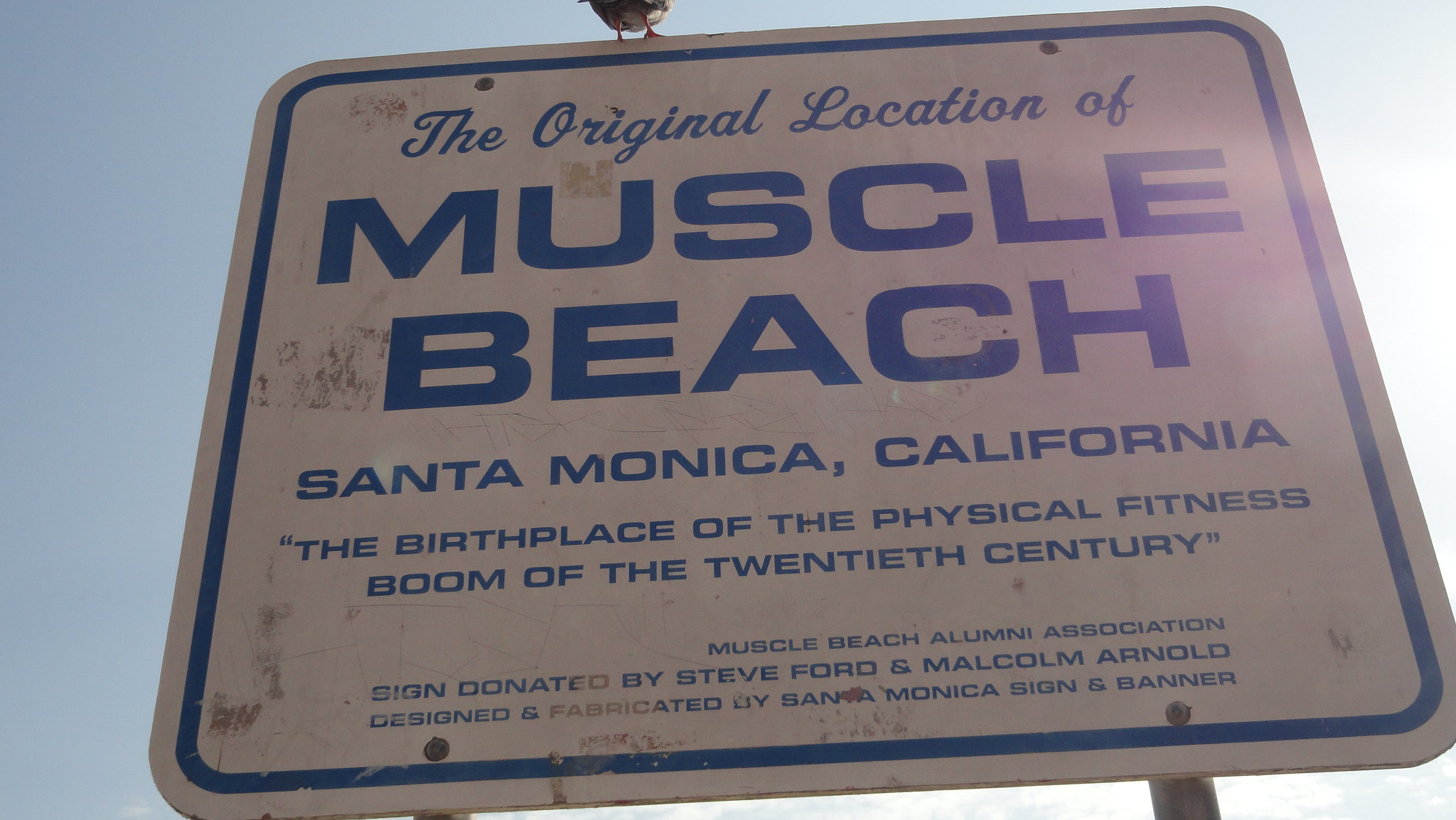The image showcases a weathered metal sign situated outdoors at the original location of Muscle Beach in Santa Monica, California, renowned as the birthplace of the physical fitness boom of the 20th century. Central to the image, the sign prominently features blue text on a slightly distressed white background, with a blue stripe along its edges. The text reads: "The original location of Muscle Beach, Santa Monica, California, the birthplace of the physical fitness boom of the 20th century. Muscle Beach Alumni Association. Sign donated by Steve Ford and Malcolm Arnold. Designed and fabricated by Santa Monica Sign and Banner." Perched atop the sign is a partially visible bird, adding a touch of nature to the scene. The sky behind is light blue with scattered white clouds, suggesting the image was taken in the middle of the day on the beach. The colors evident in the image include light blue, dark blue, white, brown, gray, and orange. The overall composition centers on the sign and its historical significance.